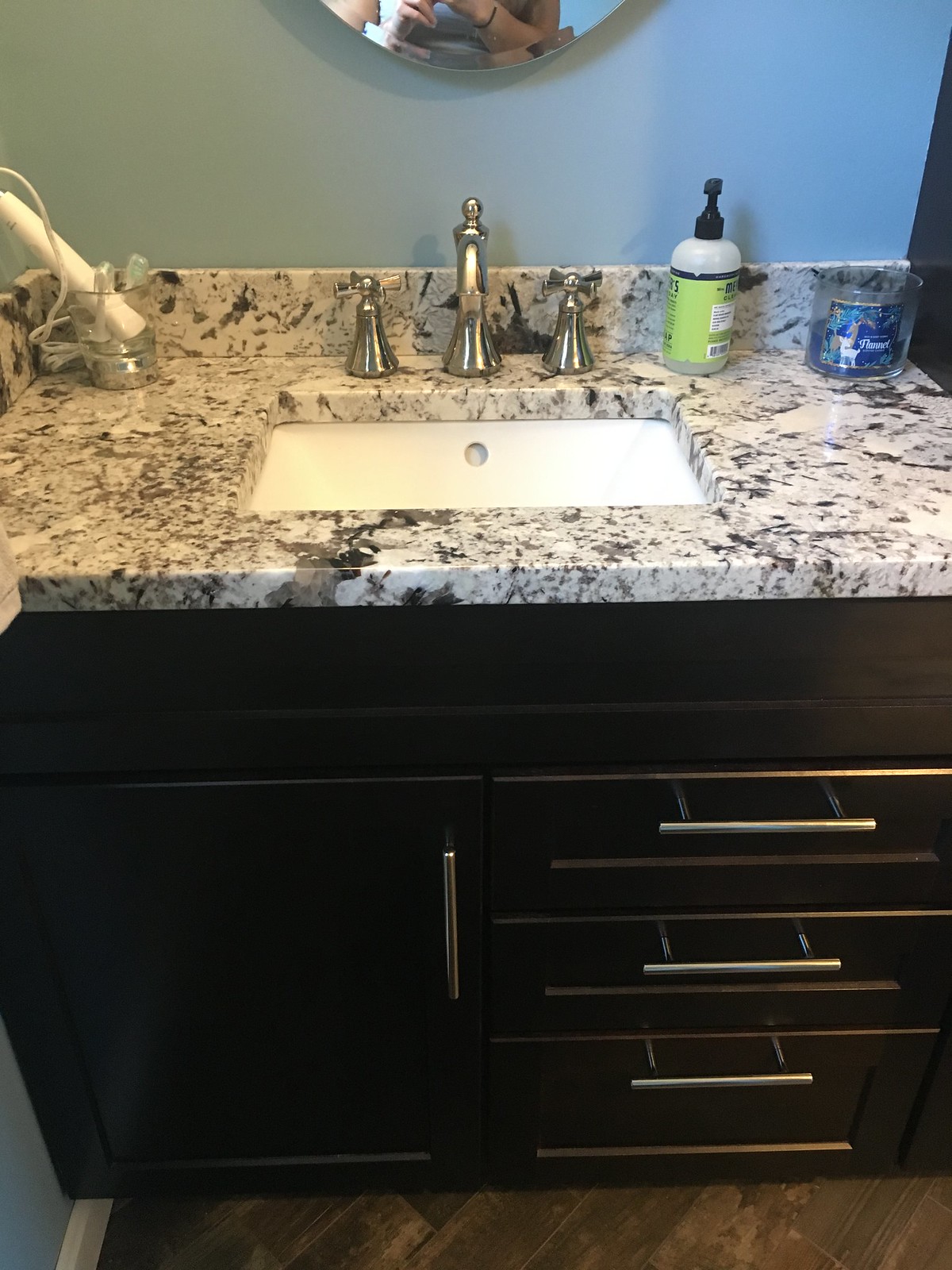This color photograph showcases a modern bathroom sink area with meticulous detail. The sink itself is crafted from white marble adorned with elegant black and gray swirls, resting atop a base that is either black or a very dark coffee color. Below the sink are three drawers featuring sleek, horizontal silver metal handles, and a cabinet door with a vertically mounted, shiny silver handle. The bathroom walls are painted a calming shade of blue, complementing the clean, sophisticated design of the sink area.

The white, undermount sink is paired with a shiny silver faucet, flanked by two matching faucet handles. Above the sink hangs a frameless oval mirror with a beveled edge, reflecting a woman taking a picture; she is identifiable by the black band on her hand. The countertop holds a few bathroom products, including soap, adding a touch of everyday life to this polished setting.